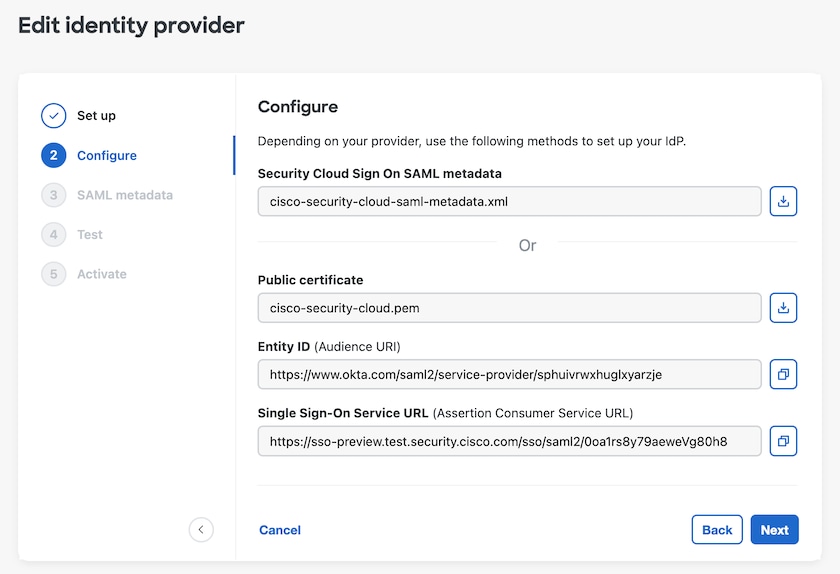Screenshot of Cisco Networking Device Configuration Interface for Website Security Settings

The image depicts the configuration interface of a Cisco networking device intended for the setup of identity provider (IDP) settings for website access. The interface is displayed on a light gray background, featuring a prominent white box that contains various configuration options.

At the top left corner, outside the white box, bold black text reads "Edit Identity Provider." Inside the white box, a vertical menu column on the left lists several options: Setup, Configure, SAML Metadata, Test, and Activate. The 'Setup' option is marked with a white circle and a blue checkmark, indicating it is completed. The 'Configure' option is highlighted in blue with a blue circle containing a white number 2, denoting it as the current active menu. The remaining options, SAML Metadata, Test, and Activate, are in light gray, indicating they are not yet accessible.

In the top center of the white box, large black text displays "Configure," followed by an instructional sentence in smaller text: "Depending on your provider, use the following methods to set up your IDP." Below this, several dialog or option boxes are presented, labeled with terms relevant to authentication and security configuration, including Security Cloud Sign-On, SAML Metadata, Public Certificate, Entity ID, and Single Sign-On Service URL.

At the bottom center of the white box, blue text provides a "Cancel" option, while the bottom right corner features navigation buttons. A white button with blue text labeled "Back" allows users to return to the previous step, and a blue button with white text labeled "Next" proceeds to the next configuration stage.

This detailed interface is intended for administrators who understand these settings and can configure them appropriately to ensure secure website access through the Cisco device.